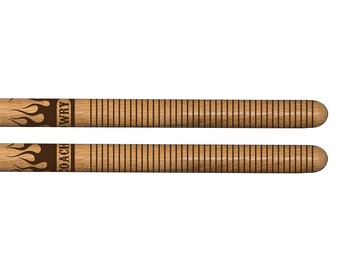The image depicts two wooden cylindrical dowels, resembling the handles of drumsticks, arranged horizontally parallel to each other with a slight gap between them. Both dowels are crafted from light-colored wood and feature identical carvings: a series of darker wood lines running along their length. The handles each have a rounded tip on the right side. At the upper portion of the dowels, there is a decorative dark brown flame pattern wrapping around them. Below the flames, there are partially visible words, with one dowel displaying "O-A-C-H" and the other "W-R-Y." The image is cropped, cutting off the dowels on the left side, creating an impression of an incomplete view. Despite the small size of the image, the craftsmanship and detailing are clear, showcasing the intricate design of these objects.